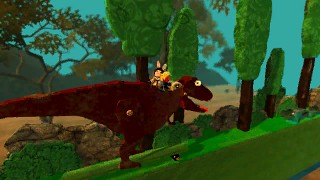The scene depicts a cartoon-style image reminiscent of vintage video game graphics, characterized by blocky, low-resolution elements. Central to the image is a brown, T-Rex-like dinosaur with a slightly flattened, 3D look similar to wooden blocks. The T-Rex, which has a long, brownish-red tail, is shown in a side profile facing to the right, with a red tongue extended from its open mouth and a googly, yellow eye. Perched on the dinosaur's back are three small characters, one notably sporting large yellow bunny ears. The dinosaur is ascending a steep, 45-degree incline covered in bright green grass. The background features a tealy blue sky and a variety of green trees, with dark brown trunks. Additionally, a dark wall appears in the image, along with a small boulder and additional foliage. Towards the foreground, the trees appear sketched, adding to the image's stylistic, whimsical nature.